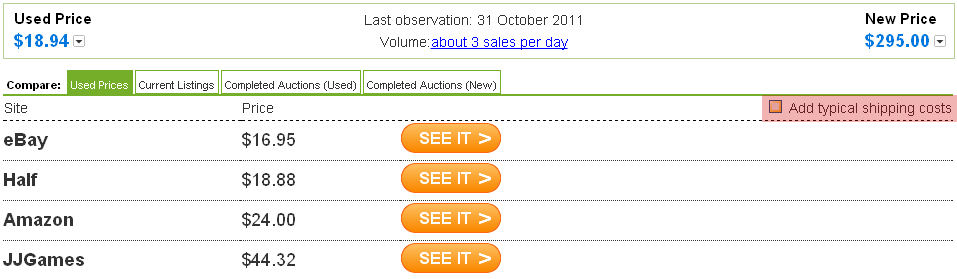This detailed screenshot showcases a price comparison website featuring both used and new product prices. The website, set against a predominantly white background, has a green-bordered rectangle displaying the "used price" prominently in blue at $18.94. Key details include the best observation date of October 31, 2011, and an average sales volume of approximately three per day. 

The new product price, also noted in blue, is significantly higher at $295. The comparison categories are divided into "used prices," "current listings," "completed auctions used," and "completed auctions new," with "used prices" being the current focus. 

Within this section, users can compare prices from different sites, which are listed as follows: eBay at $16.95, Half at $18.88, Amazon at $24, and JJ Games at $44.32. Each site listing is accompanied by an orange "see it" button on the right-hand side, providing a direct link to the respective product page. 

Additionally, there is an optional feature to "add typical shipping costs," indicated by a red-bordered checkbox, which is currently unchecked. This comprehensive layout aids users in making informed purchasing decisions by clearly presenting various price options and relevant details.